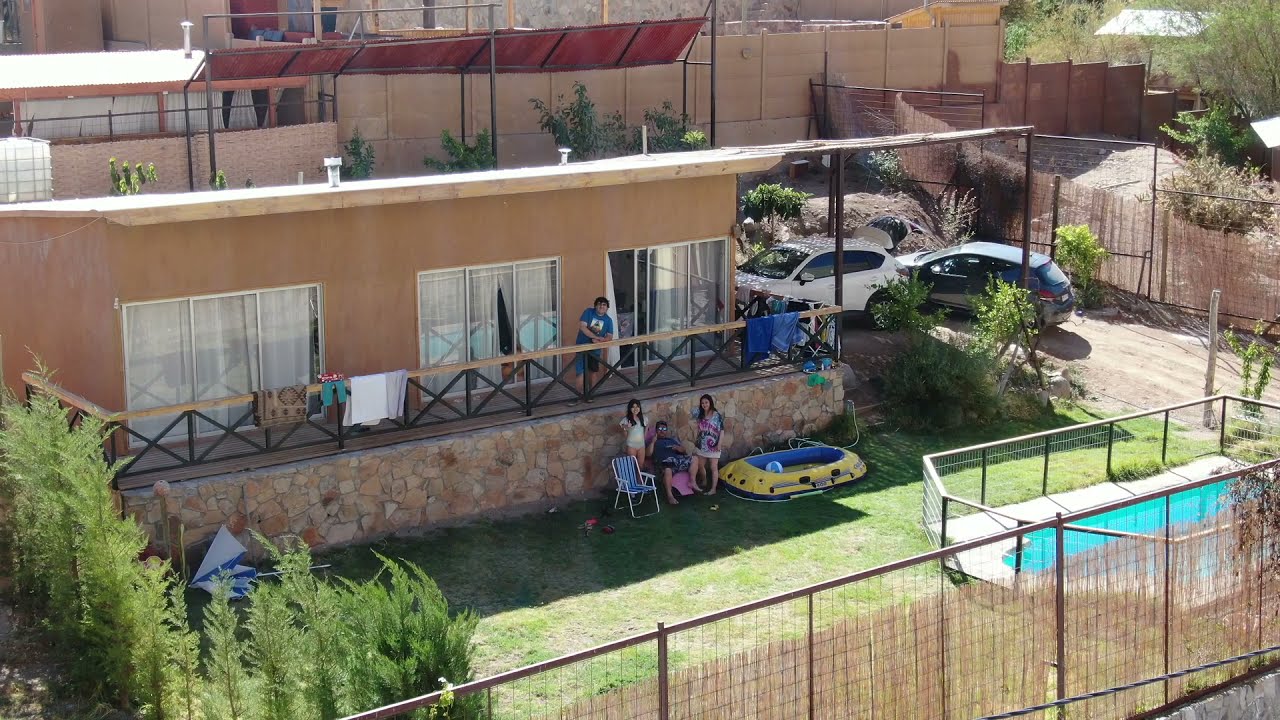This detailed color photograph, taken from a drone in landscape orientation, captures the backyard of a modest, beige one-story home built on a stone foundation. The back patio, perched higher up and secured by a steel fence with a wooden handrail, showcases a man in a blue t-shirt leaning thoughtfully on the handrail. Below him, set against the backdrop of a semi-grassy yard, a group of three women gather in the shade. One woman stands beside a blue lawn chair on the left, while another yellow and blue raft lies nearby. An empty chair quietly accompanies them. In the bottom right corner, a small swimming pool is enclosed by a chain-link fence, with an additional bamboo fence positioned at an angle in the foreground. To the right side of the home, a dirt driveway leads to two parked vehicles. Notably, other apartment buildings are visible in the background, and towels are draped over the balcony railing, contributing to the home's lived-in charm. The style of the photograph is representational realism, focusing on everyday life and human presence.